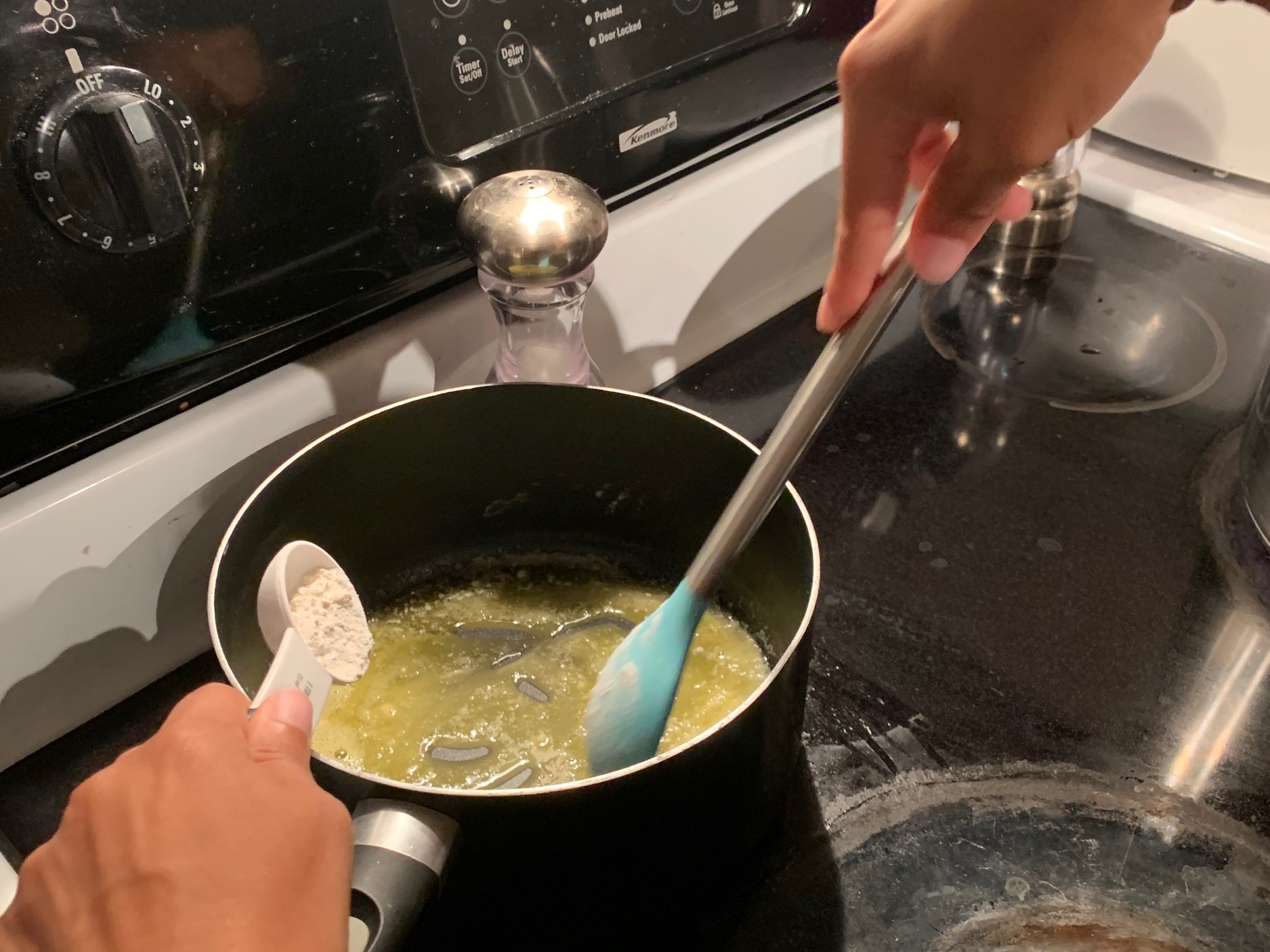A ceramic-top range with a black cooking surface and white base takes center stage in this image, clearly in need of a thorough cleaning. The stove's condition is evidenced by splattered residues, particularly around the unused burner in the foreground. At present, a nonstick saucepan sits on a burner that's switched off, its dial visible in the frame. A person's hand, potentially female given the faint pink hue on the fingernails, is seen poised over the saucepan, holding a tablespoon presumably filled with flour, ready to be added to the melted butter in the pan. Alongside, a stick-free spatula lies in wait for stirring. A salt grinder rests nearby, signifying that seasoning might be a subsequent step in what appears to be the preparation of a sauce. The scene combines elements of culinary activity with an urgent call for cleanliness.